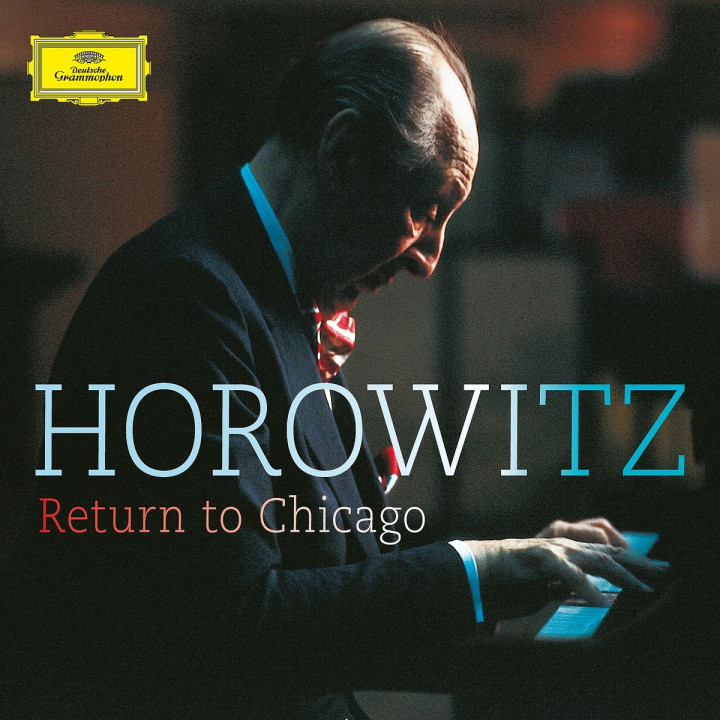This vibrant and intricate album cover features a full-color, indoor photograph of an elderly man in his late 60s or early 70s, meticulously attired in a dark blue suit, white dress shirt, and a red and white bow tie. Seated at a piano, the man, who is mostly bald with neatly combed hair over his ears, is captured in profile from his right side with his head bowed and nearly closed eyes focused intently on the piano keys beneath his hands. The image exudes a sense of deep concentration and musical engagement.

Prominently displayed across the lower middle portion of the cover in a bold, light blue, white, and dark blue Times New Roman-like font is the name "Horowitz," signifying the legendary pianist Vladimir Horowitz. Just below his name, written in a smaller, gradient red-to-pink font, are the words "Return to Chicago," announcing his much-anticipated performance or comeback. The top right corner features a decorative, Victorian-style yellow label with intricate white designs and an illegible logo or text, which adds a vintage charm to the piece. The background, composed of impressionistic cityscape elements, includes vertically aligned gray, blue, and red rectangles along with an orange sunset, contributing to the nostalgic and artistic aesthetic of the album cover.